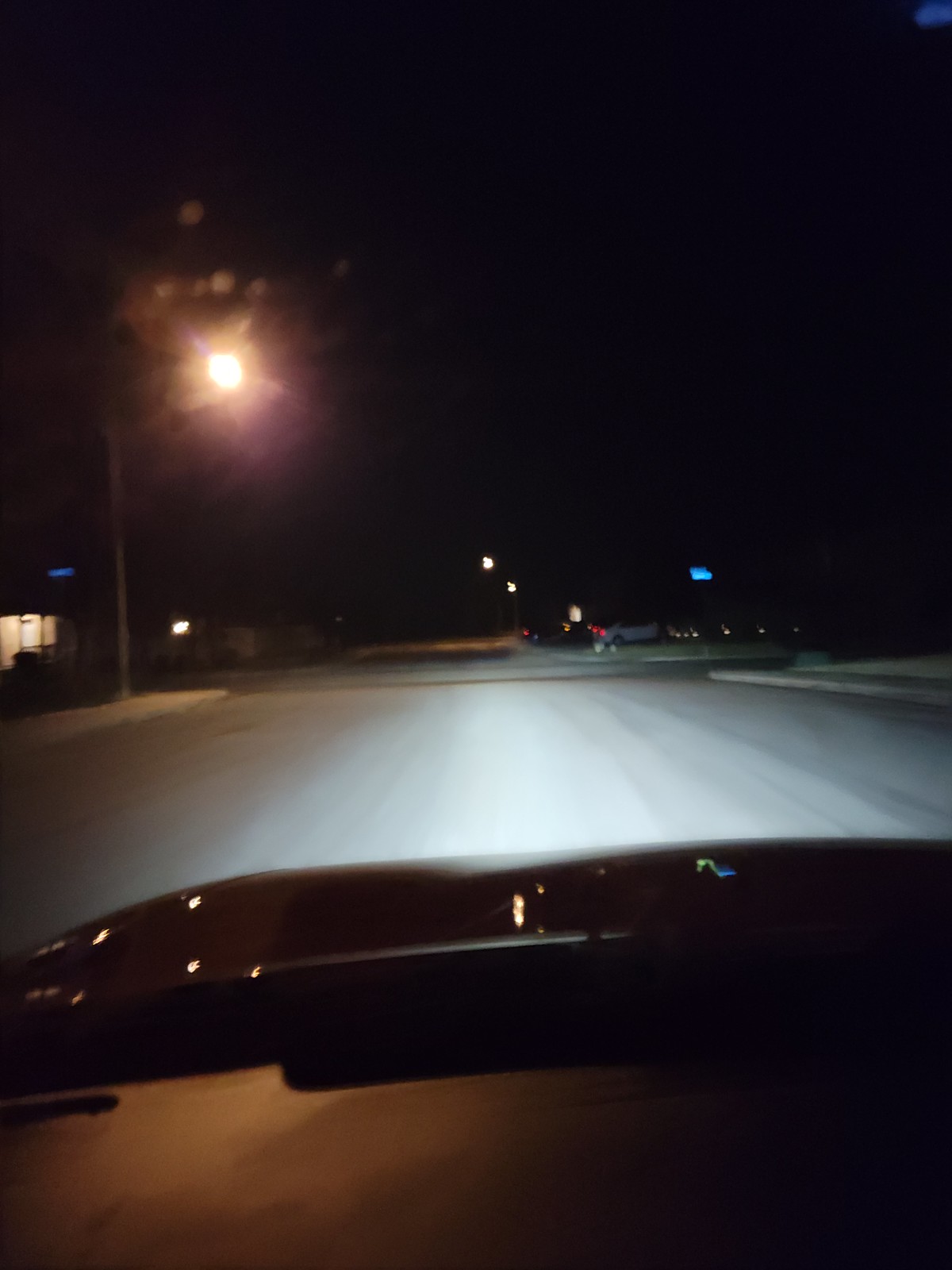The image captures a nighttime scene of a quiet neighborhood road approaching an intersection. Several cars are parked in a parking lot, all illuminated by a bright street light, which casts stark shadows on the pavement. The darkness of the night sky contrasts with the scattered street lights glowing in the distance. The viewpoint includes the black windshield and hood of the car from which the photo appears to be taken, revealing a black dashboard inside the vehicle. Blue-topped street signs are visible along the road, adding a touch of color to the otherwise muted hues of the scene. A single house is situated on the corner, emphasizing the stillness and solitude of the moment. The absence of moving vehicles on the road underscores the late hour, suggesting it is likely in the middle of the night.